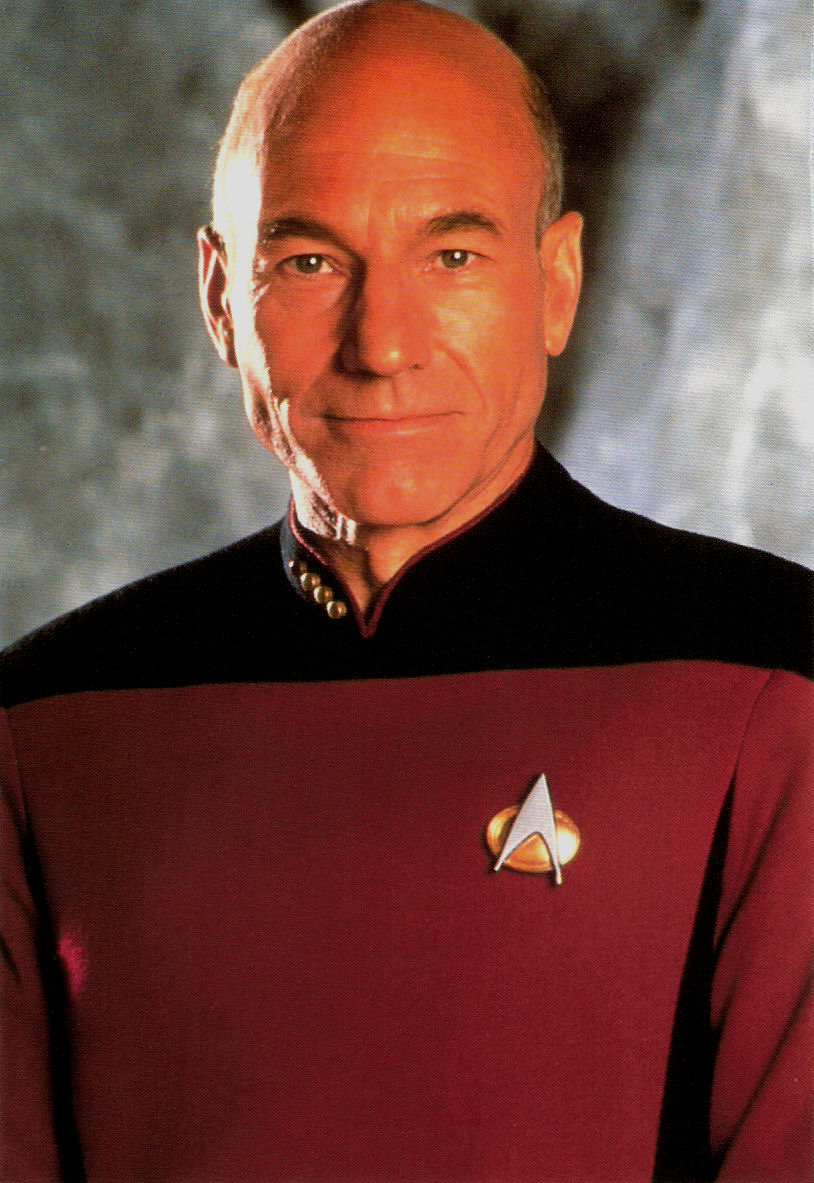The image showcases Captain Jean-Luc Picard from Star Trek, portrayed by Patrick Stewart. He is a white male with a balding head, revealing some hair at the sides, and pronounced brown eyebrows over his brown eyes. His facial expression suggests a slight smile. He is attired in a distinctive Starfleet uniform: a burgundy-red top with a black upper section and a small emblem on the right side of his chest, featuring an orange oval and an arrow-like metallic design. The uniform's collar on the left side displays four metallic dots. The background is a blurred, faded gray wall, subtly shadowed behind his head. This close-up shot focuses on his upper half, capturing his direct, almost piercing, gaze toward the viewer.